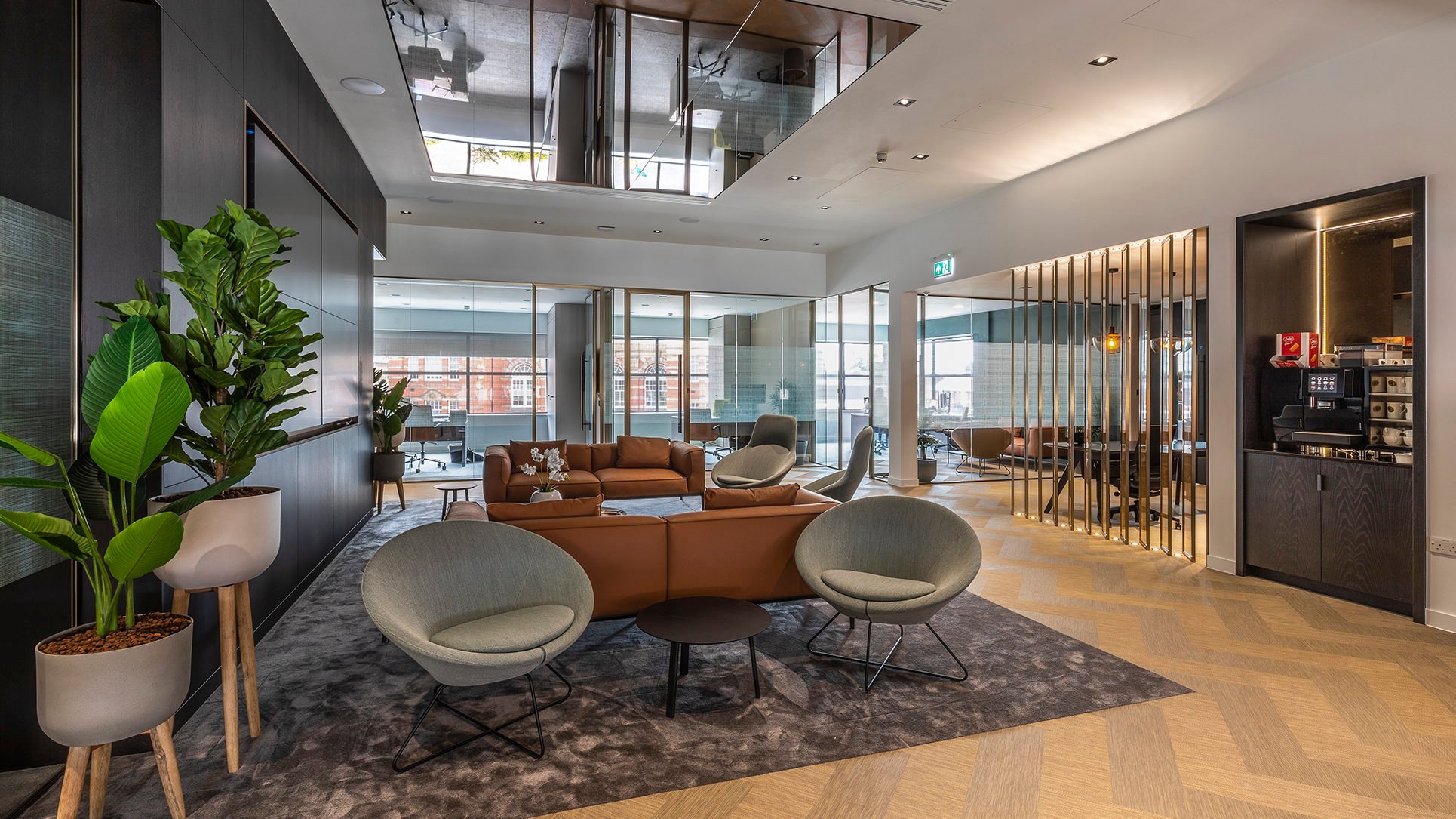This high-quality photograph showcases a modern office lobby characterized by a welcoming hospitality area, ideal for waiting on appointments. The flooring features a visually striking chevron pattern in light and dark wooden shades, which might be actual wood or a wood-look vinyl. A sizable area rug anchors a seating arrangement in the center, comprising two large brown leather sofas facing each other, flanked by several round, modern grey chairs. A sleek coffee table sits in the middle of this cozy setup. On the right, a dark wooden coffee station—with its coffee machine, mugs, and Biscoff cookies—beckons visitors for a refreshment. To the left, two lush green potted plants grace stools, contributing to the fresh and inviting ambiance. The space is illuminated by downlights and features extensive large glass windows, enhancing the airy feel. Additionally, the ceiling boasts a striking mirrored surface, adding to the modern, sophisticated atmosphere.